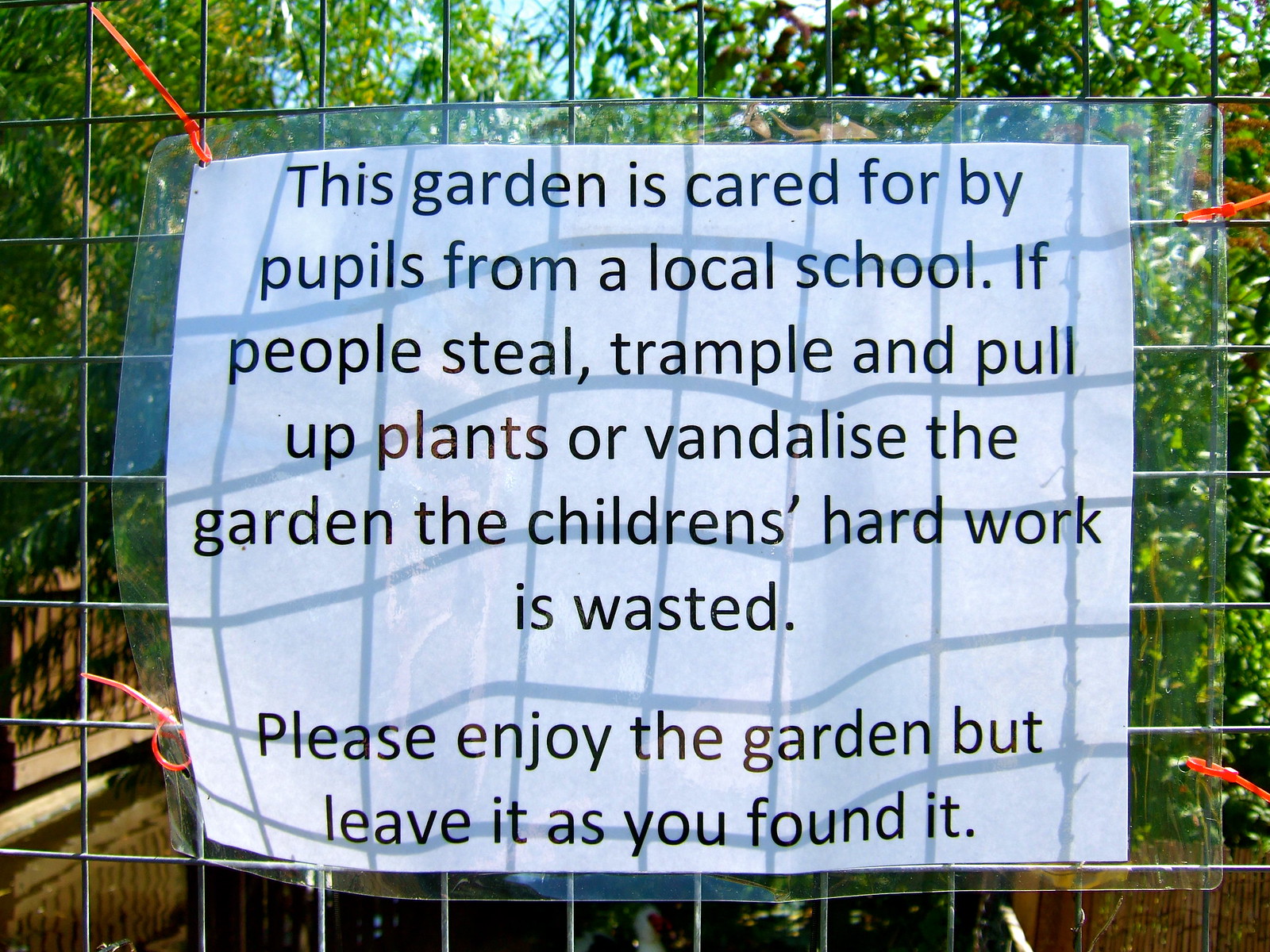This photograph shows a white paper sign laminated in clear plastic, zip-tied to a sturdy metal fence of thin horizontal and vertical bars, rather than chain-link. The sign's text is in black sans-serif font and reads: "This garden is cared for by pupils from a local school. If people steal, trample, and pull up plants or vandalize the garden, the children's hard work is wasted. Please enjoy the garden, but leave it as you found it." The plastic sleeve of the sign appears slightly warped, particularly on the lower left side. The sign is secured with red (or possibly orange) zip ties at each corner. The background reveals abundant greenery with trees, wooden fences, and potentially some bamboo fencing, indicating a lush, well-maintained garden area. The photo appears to be taken on a sunny day, as there is a noticeable reflection on the sign.